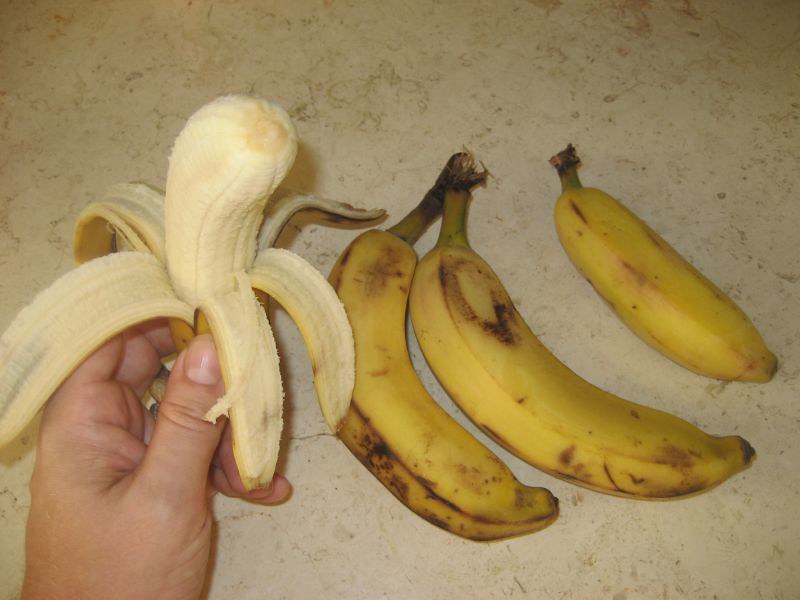In this detailed photograph, a light-skinned hand—possibly Hispanic or Caucasian—adorned with a subtle gold ring, delicately holds a partially peeled banana, its untouched fruit invitingly fresh. Surrounding the hand, amid a marbled countertop that showcases a blend of white and cream hues accented by subtle flecks, are three additional bananas. Of these, two are conjoined at the stem, resting horizontally. Beside them lies a smaller, notably straighter banana. Despite minor bruising on their peels, all bananas appear edible, and the exposed fruit of the peeled banana reveals no blemishes. The scene captures a simple, everyday moment with rich textural and compositional detail.